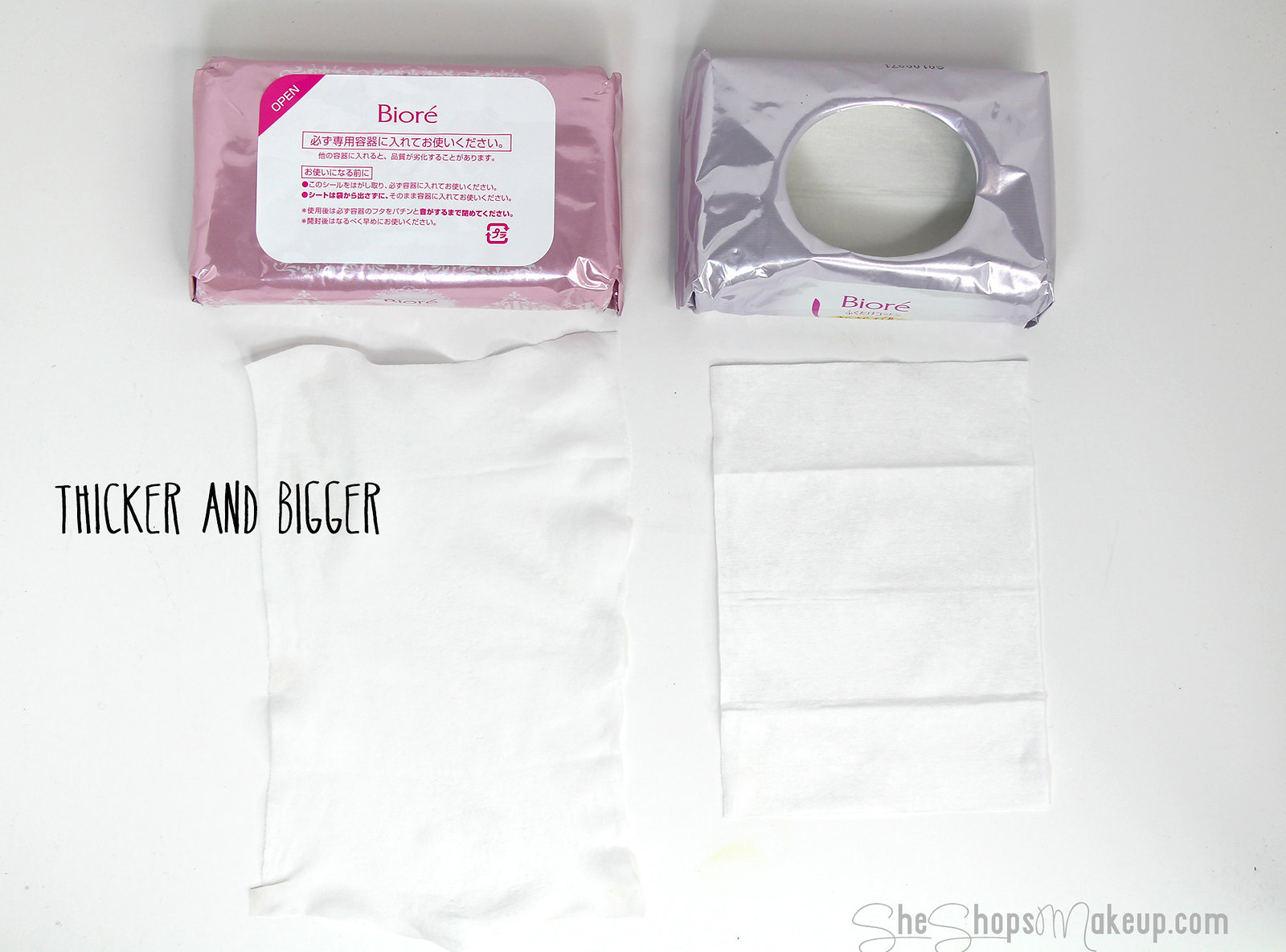This image is an advertisement showcasing two Biore facial cleansing wipe packets on a white surface. On the left side is a larger, pink, shiny foil packet labeled "Biore" with an accent and some Chinese writing, with a prominent text stating "thicker and bigger." On the right side is a smaller, silver (or light purple) shiny packet, also branded as Biore with similar Chinese text. Below each packet are the respective wipes, with the left one visibly larger and the right one slightly smaller. This side-by-side comparison illustrates the difference in size and possibly thickness between the two products, with emphasis on the larger and thicker wipe from the pink packet. The bottom right corner of the image features the website "SheShopsMakeup.com."